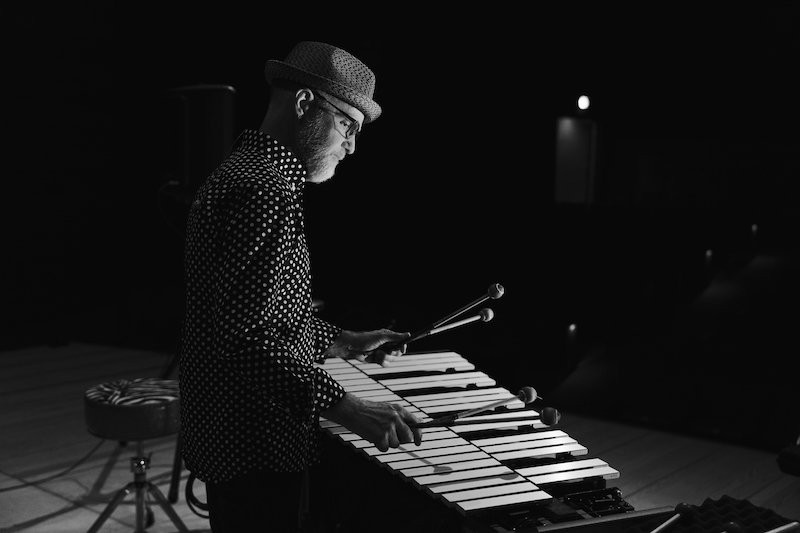This detailed black and white photograph captures an elderly man, probably in his 60s or 70s, intensely focused on playing a large xylophone on stage. The man, who has a neatly trimmed grey beard, wears a distinguished hat with a slight jazz flair, possibly a straw hat or fedora. His glasses rest firmly on his face, giving him a studious appearance. Dressed in a dark long-sleeved shirt adorned with light-colored polka dots, he rolls up the cuffs for comfort. In his hands, he skillfully holds two pairs of xylophone mallets, each with a round ball at the end, poised to strike the instrument's two-tiered layout. Below him, a small stool sits on the stage, which is enveloped in darkness except for a singular white circle of light in the distance, highlighting the performer in a dramatic fashion.